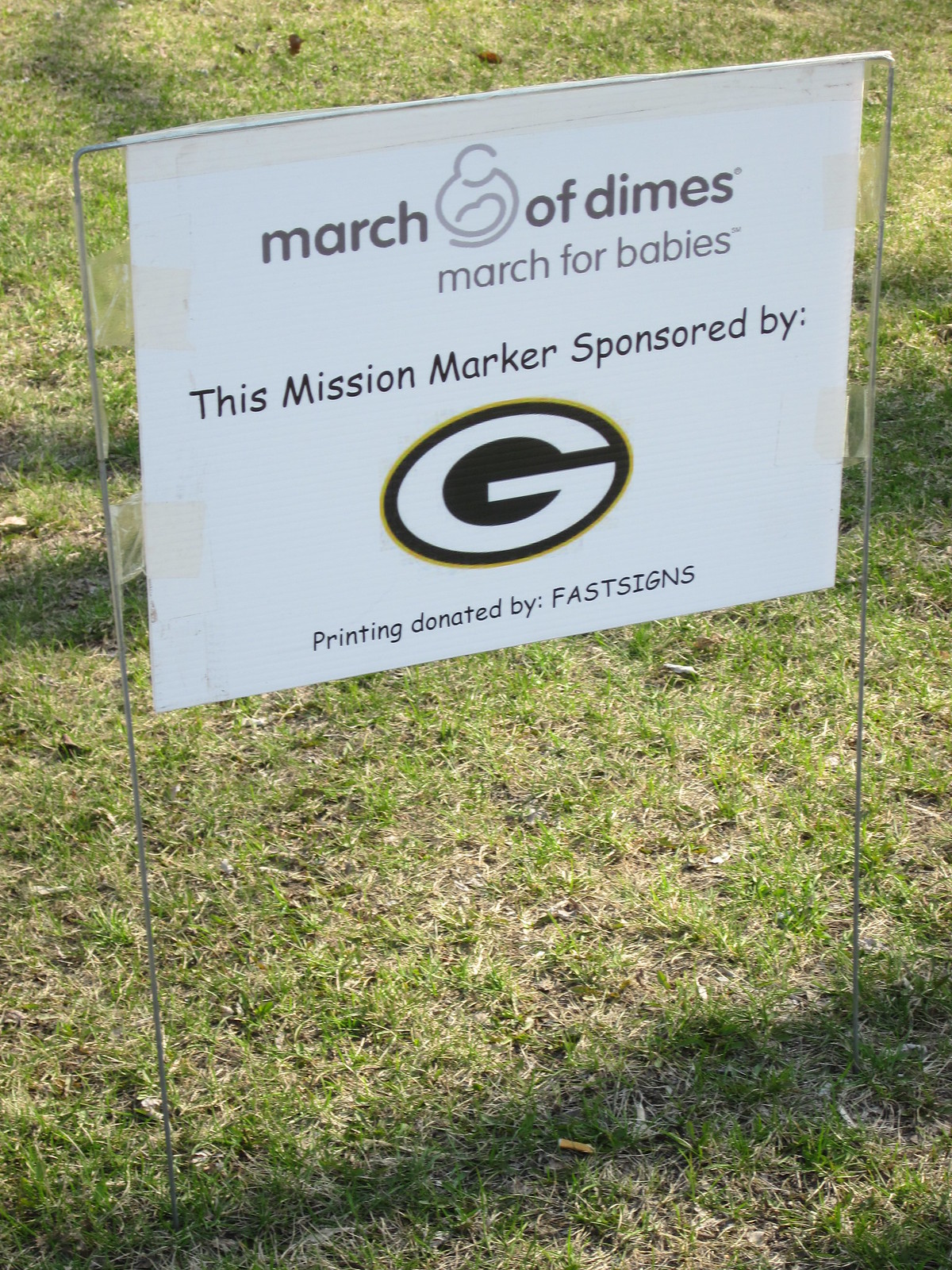This is a detailed photo of a rectangular yard sign stationed in green, well-maintained grass on a sunny day. The sign, which is white with black text, is fixed to a thin, silver metal frame using visible packaging tape. The top of the sign reads "March of Dimes, March for Babies," accompanied by a logo depicting a person holding a baby, rendered in minimalistic lines. Below this, the text states, "This mission marker sponsored by Georgia," featuring the Georgia Bulldogs football logo, characterized by a bold 'G' with black and yellow outer rings. Further down, the sign acknowledges, "Printing donated by F.A.S.T. Signs," displayed in all capital letters. The scene is brightly lit, casting shadows from unseen trees, adding depth to the background. The sign is prominently placed, surrounded by abundant white space, making the content stand out clearly.